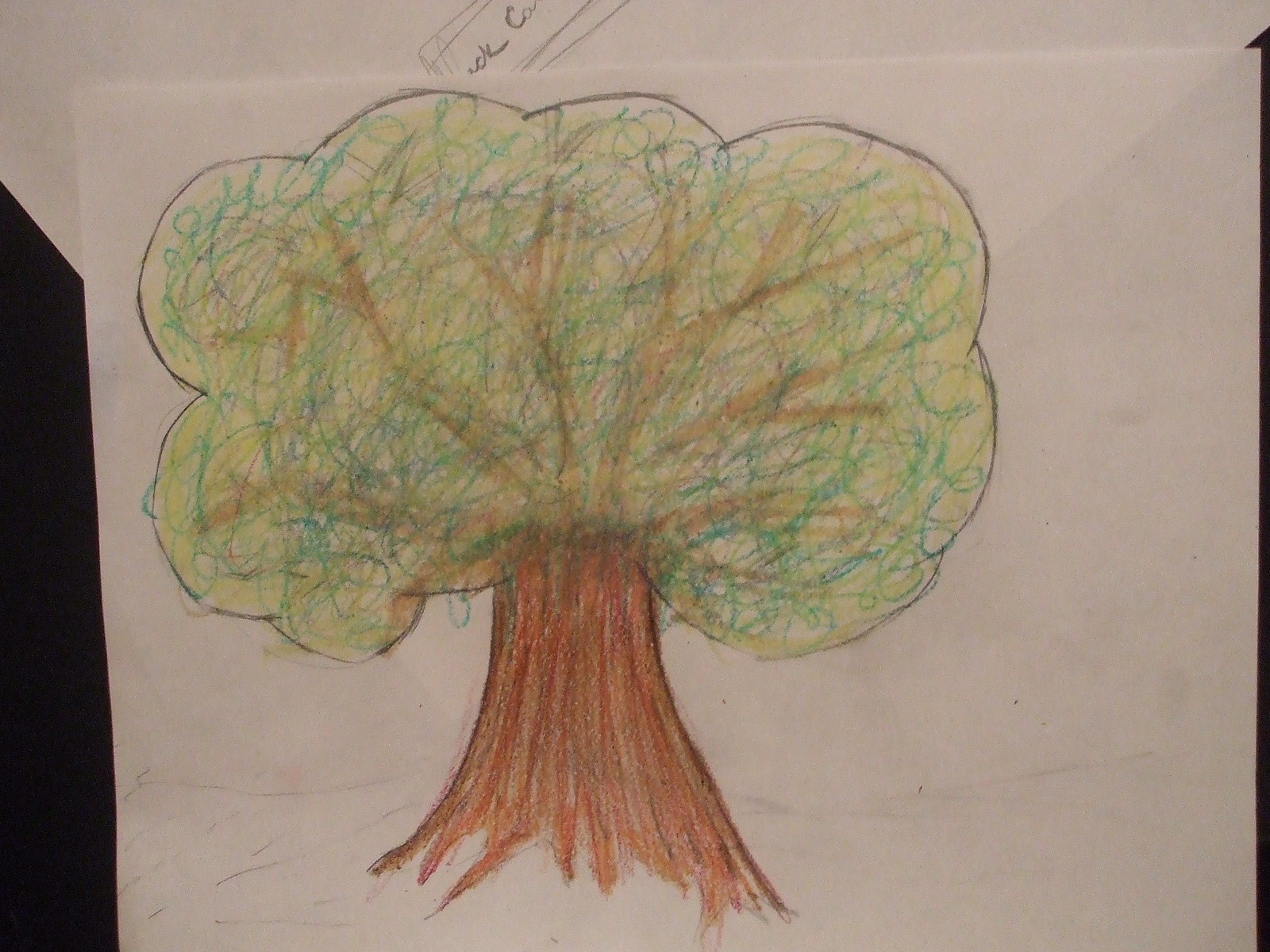This illustration showcases a tree rendered with a mix of pencil, colored pencils, and crayons. The tree's contour is meticulously outlined in pencil, while its interior is vibrantly filled with an array of hues, primarily green, yellow, and brown. The coloring technique within the tree consists of expressive scribbles, lending a dynamic texture to the foliage. Lightly sketched branches are interwoven within this colorful scribble, likely drawn with either crayon or marker to add depth. The trunk of the tree is prominently brown, filled using a crayon or marker to create a solid base. This artwork is set on a slightly off-white, lightweight construction or drawing paper, adding a subtle earthy undertone to the overall composition.